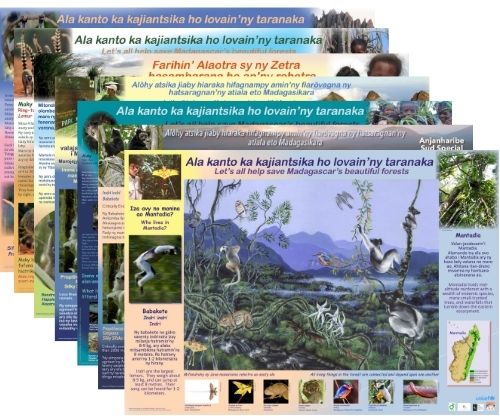The image features a series of vibrant, digitally placed posters arranged in a cascading format, partially obscuring each other. Each rectangular poster includes colorful, detailed artwork and text. The prominent front-most poster showcases an enchanting painting of a sparse forest with various animals, including monkeys hanging from tree branches. The scene is rich in hues of blue, green, grey, and light peach. 

At the top of this lead poster, there is a series of words in a foreign language: "Allah, Kanto, Ka, Kajianski ka, Ho, Loven, Nai, Taranka". Beneath this, a message in English reads, "Let's all help save Madagascar's beautiful forests." Additional elements on this poster include various photographs of wildlife situated in the corners and supplementary text and images scattered throughout. A similar theme of forest conservation and vibrant nature continues across the partially visible posters behind it, creating a layered effect.